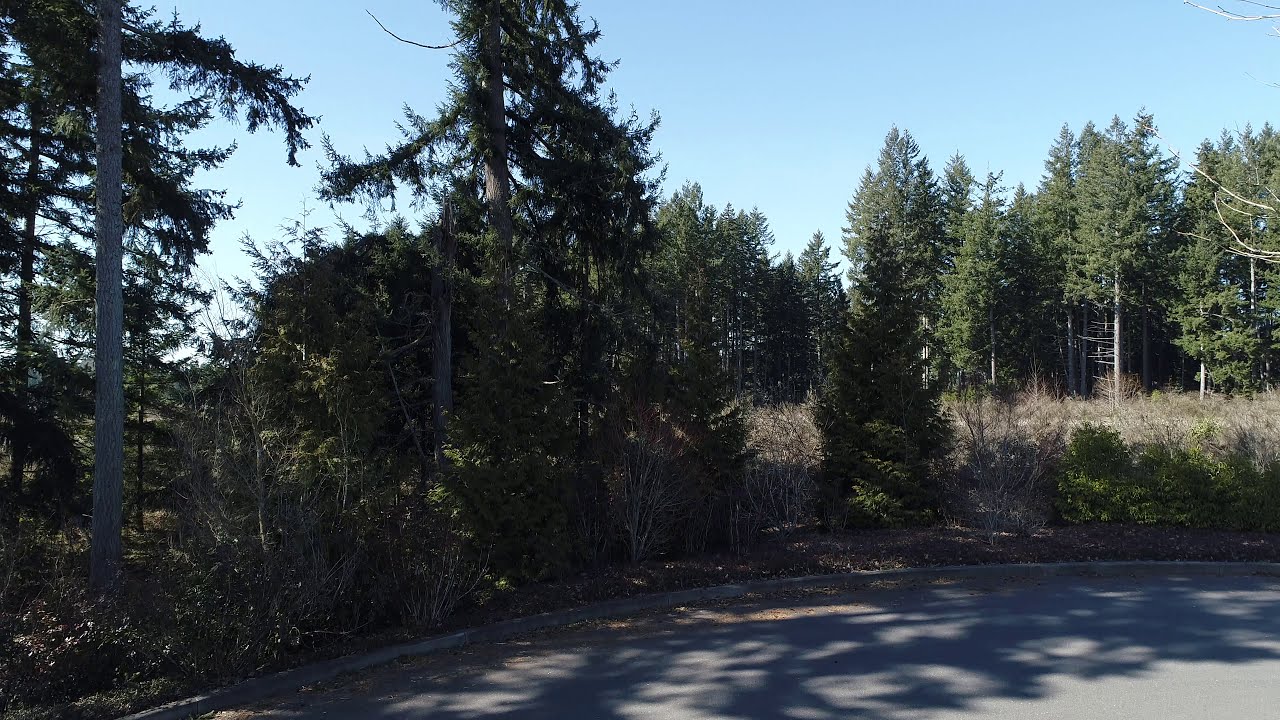The photograph captures a tranquil, scenic spot during the daytime, situated at the end of a dead-end road shaped like a cul-de-sac. The paved road, seemingly off the beaten path, is enveloped in the shadows cast by a small grouping of pine trees and other types of trees, lending a sense of seclusion and peace to the area. The trees in the background vary in height, with some standing tall and others shorter, creating a diverse natural canopy. A small, grassy field with tall, possibly dead grass stretches beyond a walkway that cuts through a couple of bushes, leading into the lightly wooded area. The tops of the pine trees are lush and green, mingling with some dead leaves. The ambient sunlight filters through the leaves, projecting a mix of light and shade that enhances the serene atmosphere of this out-of-the-way, picturesque location.